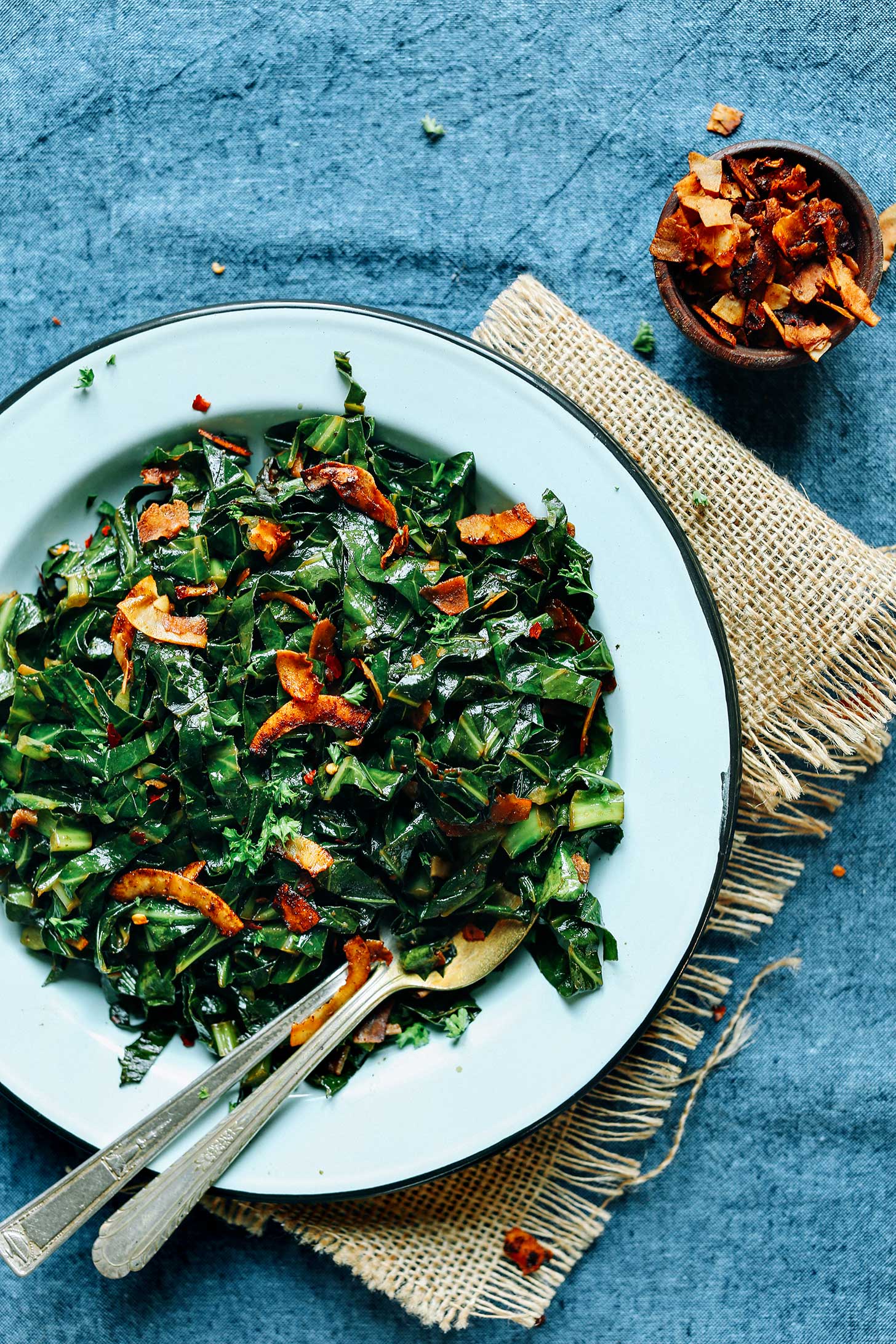This image showcases a white ceramic dish with a dark green border, elegantly arranged on a burlap-textured tan napkin atop a dark blue tablecloth. The dish appears to be a leafy green salad, accompanied by chopped grains and vibrant orange pieces, possibly seasoned with an orange sauce or marinated. A silver fork and spoon are nestled within the salad, their handles clearly visible, with one utensil featuring a more squared end and the other a more curved one. Additionally, a small bowl containing what looks like orange flakes is situated in the background, suggesting these flakes were incorporated into the salad. The scene is further accented by a few loose flakes spread across the table, adding a touch of rustic charm to the composition, reminiscent of a carefully styled magazine culinary feature.